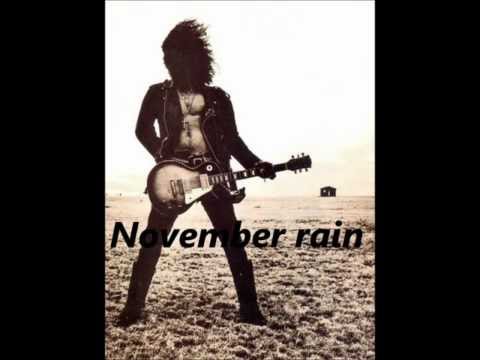In this black-and-white photograph, a man stands in an open field, holding an electric guitar at waist level. His hair appears windblown and dark-colored, adding to the image's dynamic feel. He's clad in an open leather jacket, which reveals his bare chest and a necklace, paired with black pants and tall boots. The sky above him is light gray, suggesting a cloudy day, and the field's grass appears beige, indicating a muted, grayed-out aesthetic. A small house or barn is visible in the background on the right-hand side, adding depth to the scene. Across the man's knee level, the caption "November Rain" is prominently displayed in capitalized black font, albeit slightly difficult to read due to the dark tones of the image. The composition is framed by two solid vertical black strips on either side, further emphasizing the central focus on the man and his guitar.